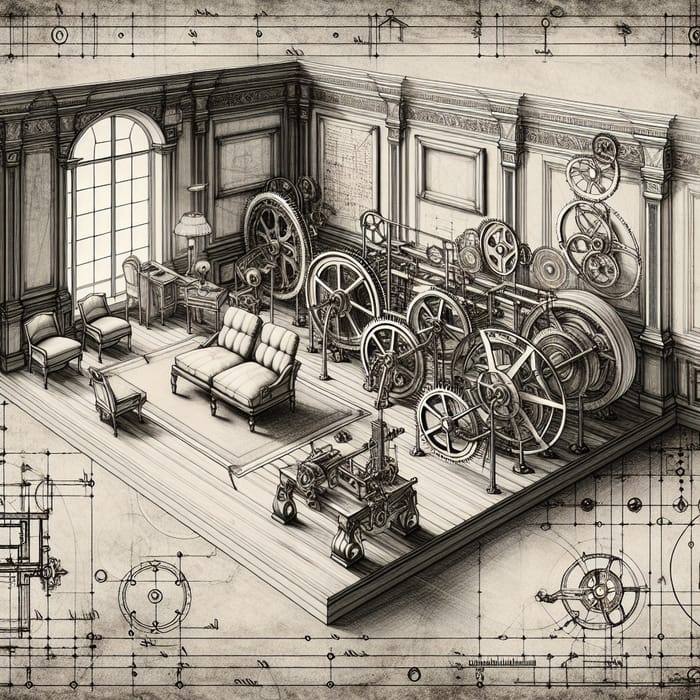The image is a highly detailed, black-and-white pencil drawing of a Victorian-style lounge or sitting room viewed from above. The room features an ornate interior with very high ceilings and tall French windows. Situated on a wooden platform, the room is divided into two distinct areas: a living room furnished with three single chairs, a loveseat, a table lamp, and a desk with a desk chair, all arranged beneath an arched, stained-glass window. The walls are intricately designed with columns that separate various panels. 

The rear section of the room is unique, showcasing an elaborate array of interlocking gears of different sizes, some stacked upon each other and several encased by a belt, suggesting they are designed to be in motion. This gear machinery stands upright along the back wall of the room. Surrounding the main illustration are technical elements, including architectural-style drawings depicting blueprints of the gears and musical lines akin to sheet music at the top, lending the image an industrial yet whimsical quality. The entire composition is done in a rectangular shape, emphasizing both artistic and technical prowess.